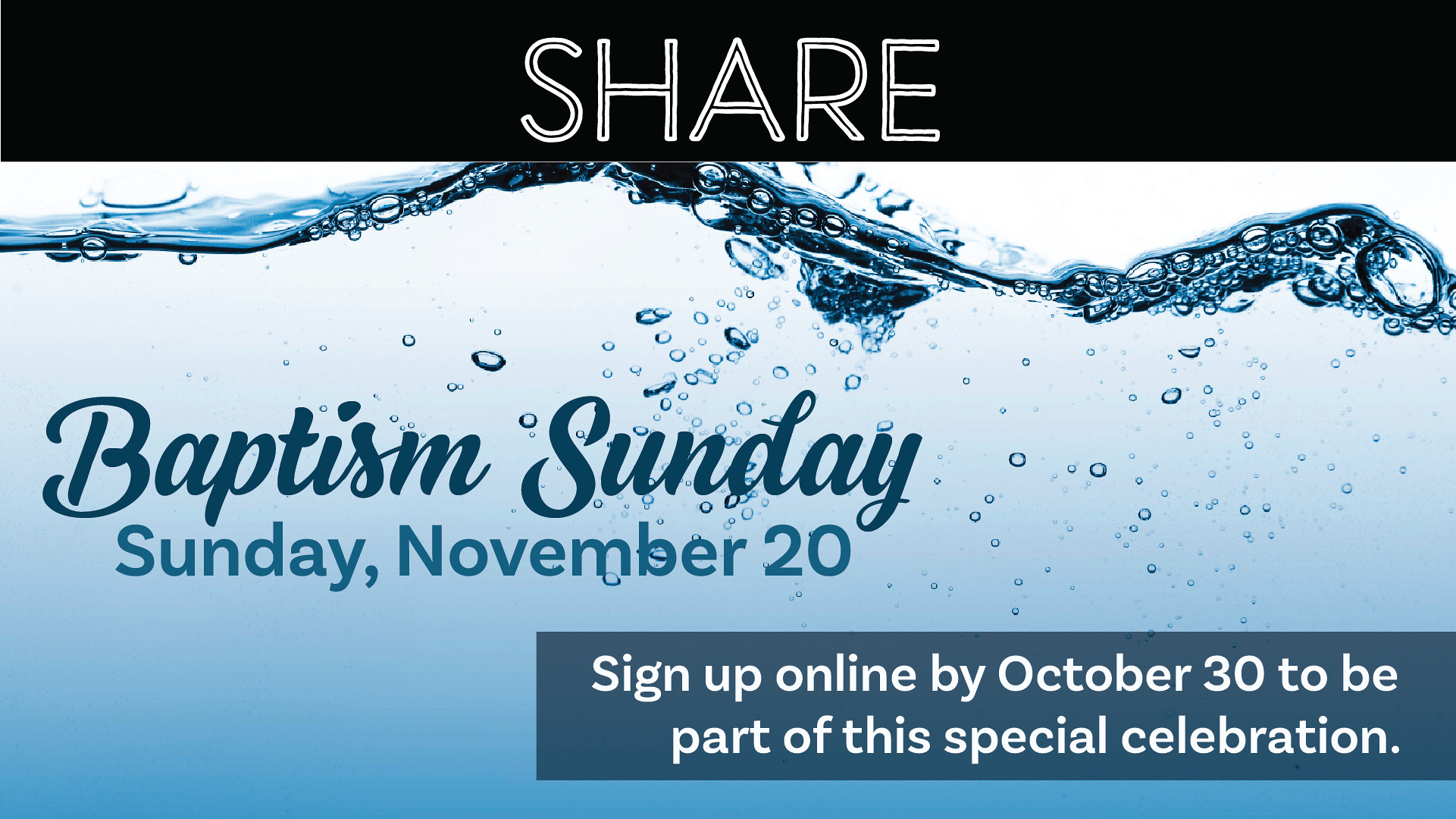The image features a prominent black bar at the top with the word "SHARE" in white, hollow lettering. Below this bar, there is a depiction of blue water, marked by dark lines and bubbles, adding a sense of movement as if viewed from underwater. In the center of the image, a light blue shaded section contains the text "Baptism Sunday" in a cursive font, followed by "Sunday, November 20th" in blue letters. At the bottom, a blue bar holds the message in white letters: "Sign up online by October 30th to be part of this special celebration." The overall design incorporates a fluid, aquatic theme to highlight the nature of the Baptism event on Sunday, November 20th, capturing the essence of the water and the significance of the celebration.